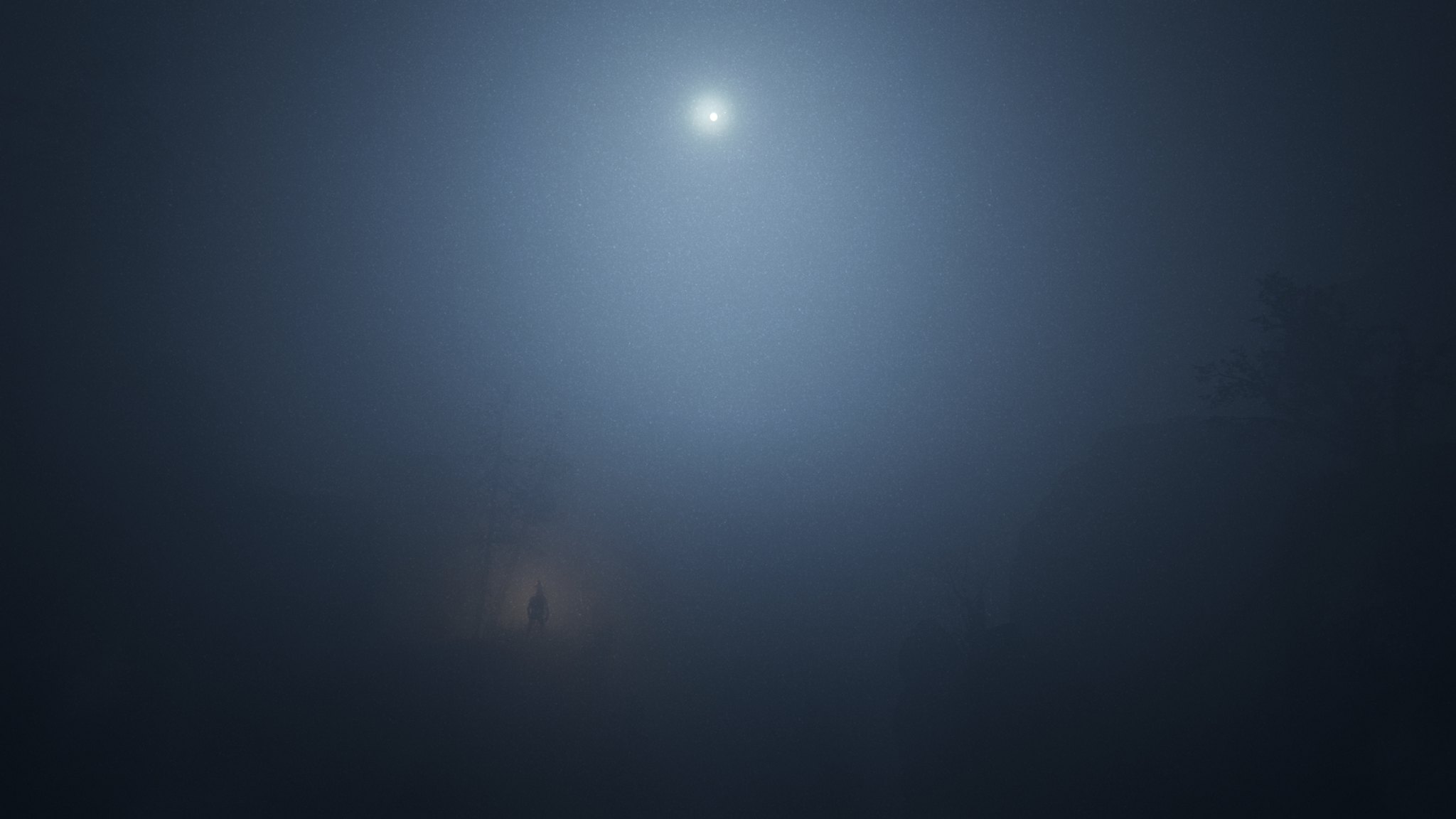In this atmospheric nighttime scene, either a photograph or a computer-generated piece of art, the focal point is a mystifying combination of light and shadow. The image is enveloped in a dreamy mist that softens the contrast between darkness and light. At the pinnacle of the composition, a small, glowing white circle, resembling the moon, casts a gentle, ethereal glow. The periphery of the image is swathed in deep black shadows that gradually lighten as they ascend towards the luminous moon. At the bottom, a mysterious silhouette, possibly of a person or an animal, stands on the ground. This figure is subtly highlighted by a faint, orange aura, adding a mystical touch to the surreal ambiance of the scene.